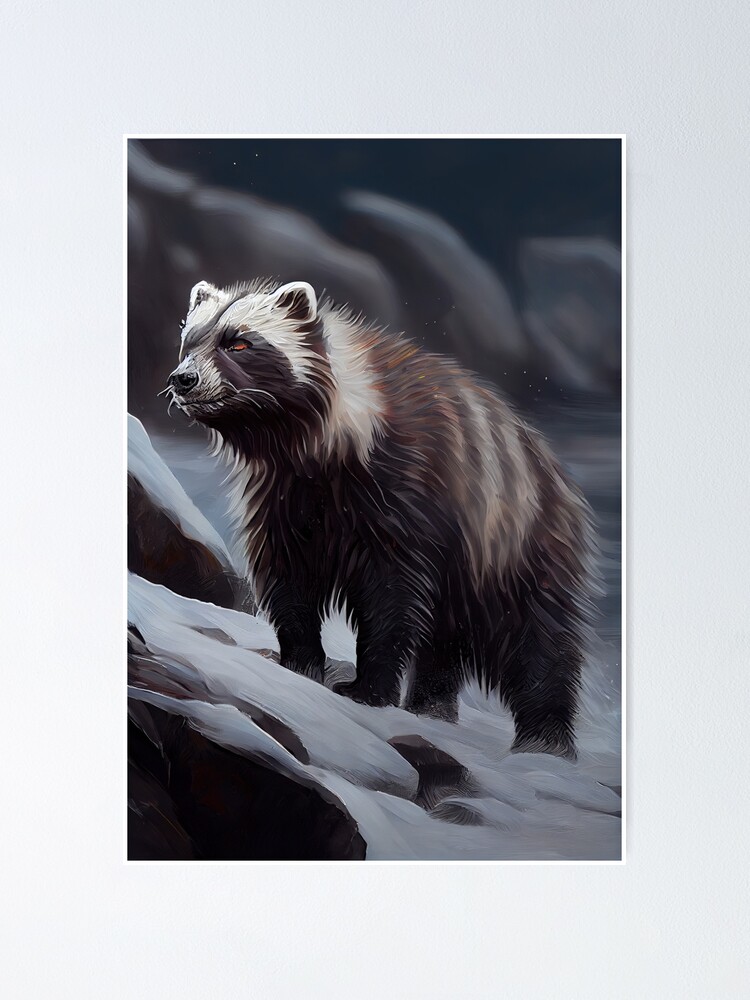The image depicts a detailed, computer-generated illustration of a bear, characterized by a facial expression that exudes seriousness and no-nonsense. This bear features a striking black and white coloration, resembling a badger, especially around its face, ears, and neck. The bear stands tall, with all four legs firmly planted on what appears to be a layer of snow-covered ground, possibly atop a gray rock. The bear's eyes are a vivid orange, adding intensity to its gaze as it looks off to the side. The background suggests a cold environment, with a hint of an evening sky, and the distant presence of mountains and rocks. The image has the aesthetic quality of an oil painting, framed centrally within a rectangle, with a gradient background that transitions from gray at the top to white at the bottom.